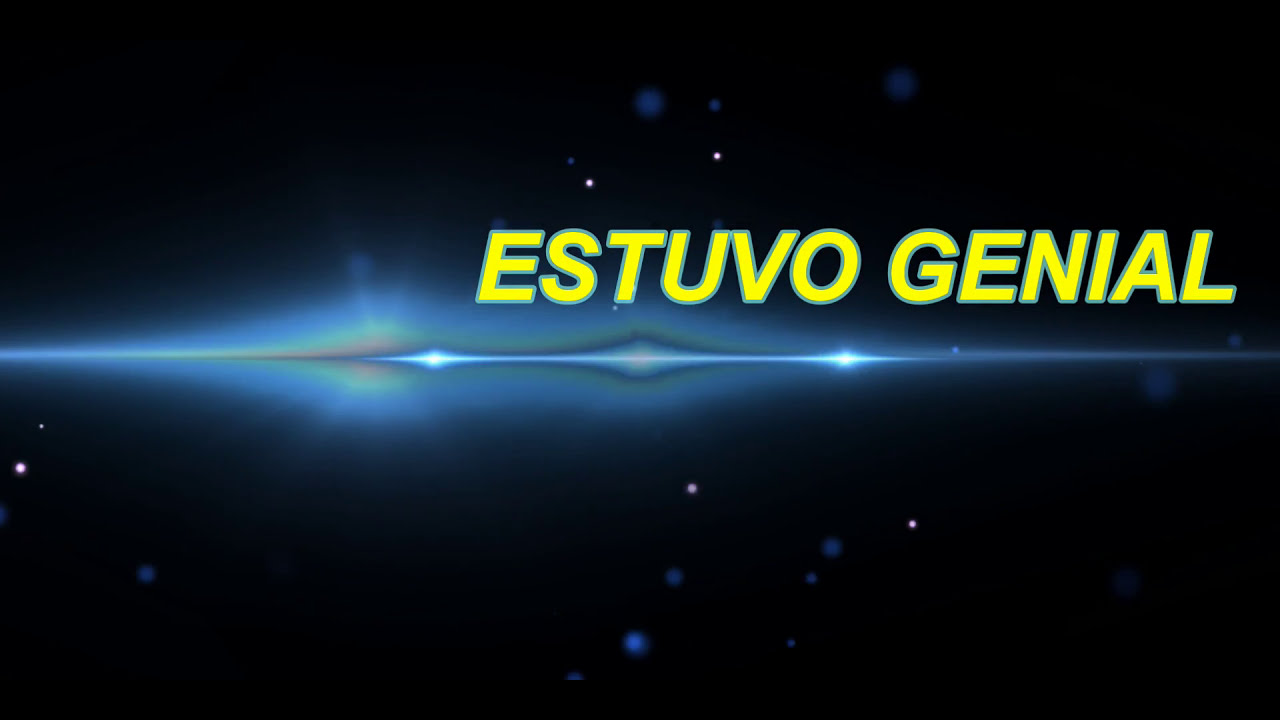The image features a wide horizontal rectangle with a predominantly black background, representing outer space. Sprinkled throughout the blackness are tiny dots of varying colors—blue, white, and purple—depicting distant stars or light sources. Cutting across the center of the image is a thin, glowing line of light blue, occasionally intensified with white to enhance its luminescence. Above this glowing line, the text "ESTUVO GENIAL" is prominently displayed in bold yellow capital letters, outlined with the same light blue hue as the line. The text aligns centrally in the upper portion of the image, with the first word "ESTUVO" placed in the center and the second word "GENIAL" slightly to the right. The background includes subtle, abstract details such as motes of light and a series of lens flares, adding to the image's cosmic ambiance.